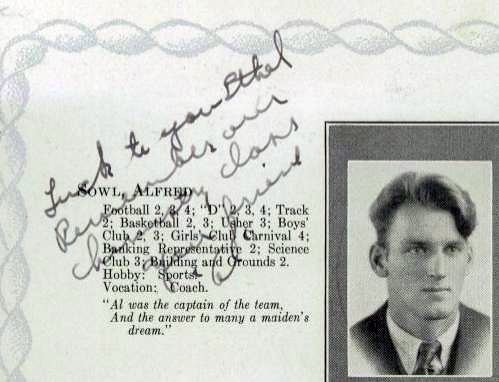This detailed caption provides a cohesive description of the image:

This is a black and white document on an off-white background, adorned with a light gray decorative frame along its top and left side. The document appears to be a bio of an individual named Scout Alfred. It lists his involvement in various activities: Football 2-3-4, D-2-3-4, Track 2, Basketball 2-3, Usher 3, Boys Club 2 and 3, Girls Club Carnival 4, Banking Representative 2, Science Club 3, Building and Grounds 2, Hobby, Sports, and Vacation Coach. There's a notable caption stating he was the captain of the team and "the answer to many a maiden's dreams." Towards the middle right is a black and white photograph of a young man enclosed in a gray and black frame. There is handwritten text overlaying the photo that reads "luck to you," with some parts written in cursive but not entirely legible. The entire image is a monochromatic palette of black, gray, and white.